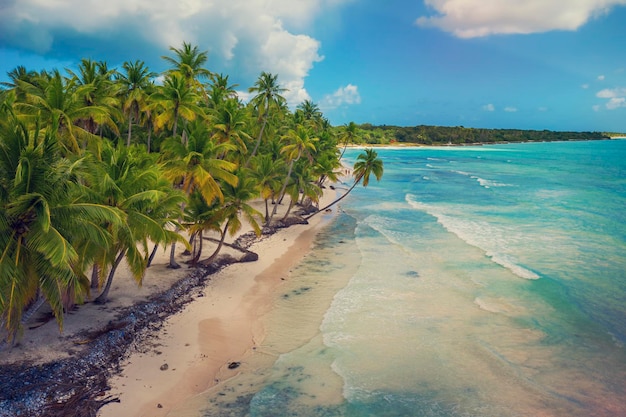This image captures a pristine, tropical beach from an overhead perspective. The majority of the scene is composed of clear, blue-green ocean water gently lapping onto a sandy shoreline. The sky above is mostly clear with a few fluffy, white clouds, casting a bright, sunny light over the serene landscape. On the left side of the image, a line of palm trees with long, slender trunks and dense, heavy fronds stretches along the shoreline, emphasizing the tropical nature of the location. One prominent palm tree arches outwards over the ocean, adding a picturesque element to the scene. There is no visible trash or industrial presence, only the natural beauty of the clean beach and lush greenery. In the background, the rest of the island or additional landmass, is densely covered with more trees, contributing to the overall impression of a tranquil, isolated paradise.